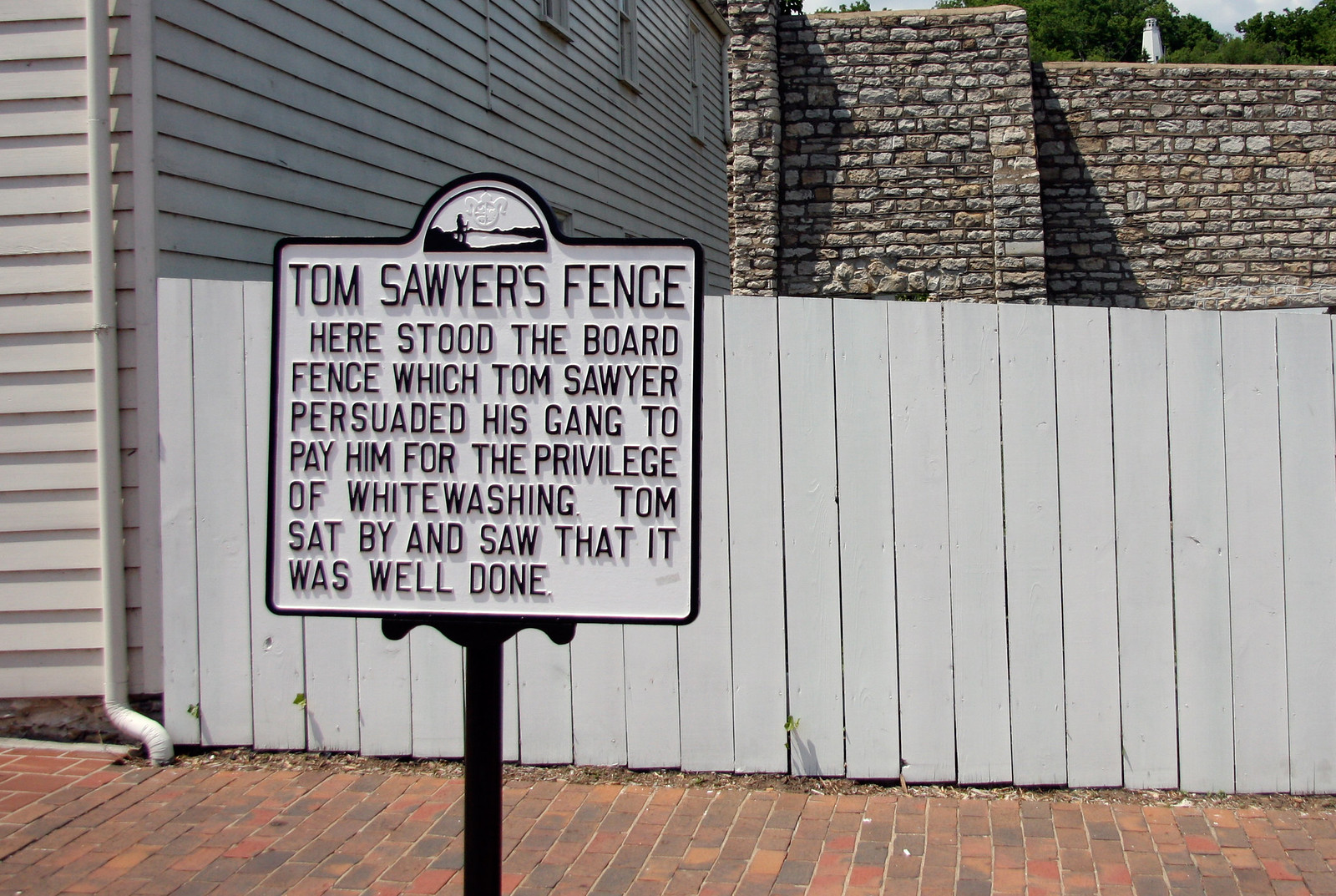The image depicts a historical sign prominently positioned in front of a classic, colonial-style whiteboard fence, which is painted and borders a cobblestone street made of red and black bricks. The sign itself is a white metal rectangle with a black outline, approximately two feet by two feet in size. It features raised black lettering that reads: "Tom Sawyer's Fence. Here stood the board fence which Tom Sawyer persuaded his gang to pay him for the privilege of whitewashing. Tom sat by and saw that it was done well."

Behind the fence stands a white-paneled building, shadowed by the sun high in the sky, which casts shadows on its roof. Further in the background, there is another building, constructed from brown and white stone, contributing to the historical ambiance of what appears to be a quaint, small-town setting. The placement of the sign, clearly intended for tourists, highlights its significance and marks the historical site with clarity and prominence.